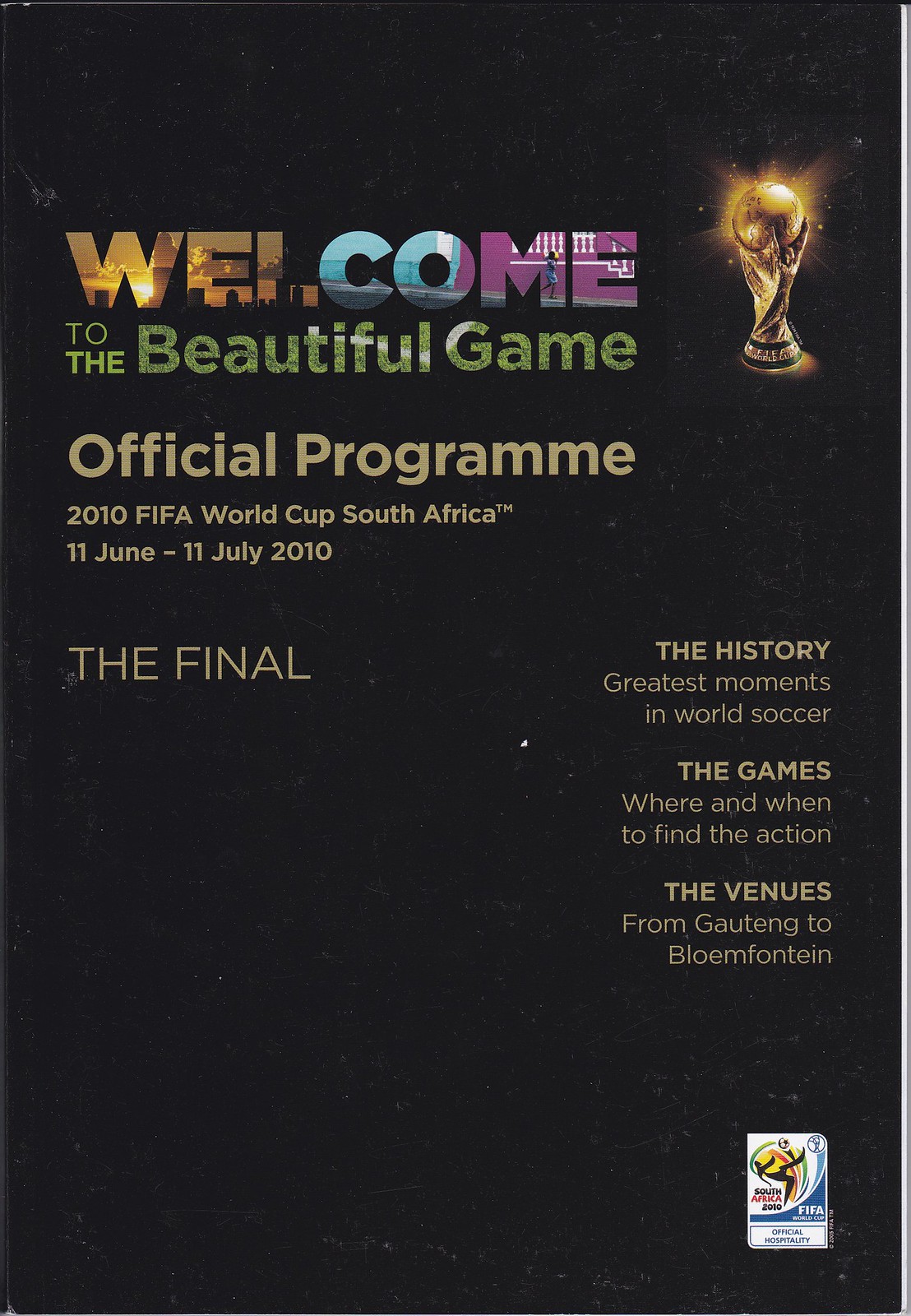This image appears to be a scan or picture of an official program for the 2010 FIFA World Cup held in South Africa. The background is a very dark brown, almost black, though parts of it appear slightly faded with age. 

In the upper right corner, there is an image of the FIFA World Cup trophy, rendered to look like it’s glowing. To the left of the trophy, the word "WELCOME" is prominently featured. The letters of "WELCOME" are creatively overlaid with various images; the "WL" forms a bluish wall-like city skyline, while the "CO" and "ME" sections are sunset images and other scenic views of South Africa. Below this, the text "to the beautiful game" is displayed, with a greenish photograph of a soccer pitch serving as the background for the words. 

Further down, in gold text, it reads "Official Program 2010 FIFA World Cup South Africa, 11 June to 11 July 2010." Below this, it mentions "The Final" and provides additional details such as "The history, greatest moments in world soccer, the games, where and when to find the action." It also lists the venues, including "from Gauteng to Bloemfontein." At the very bottom right, the official 2010 FIFA World Cup logo can be seen, marked with text that includes "South Africa 2010" and "Official Hospitality."

The overall design indicates it is a comprehensive guide to the tournament, providing insightful information about the history of the World Cup, key moments, game schedules, and venue details.